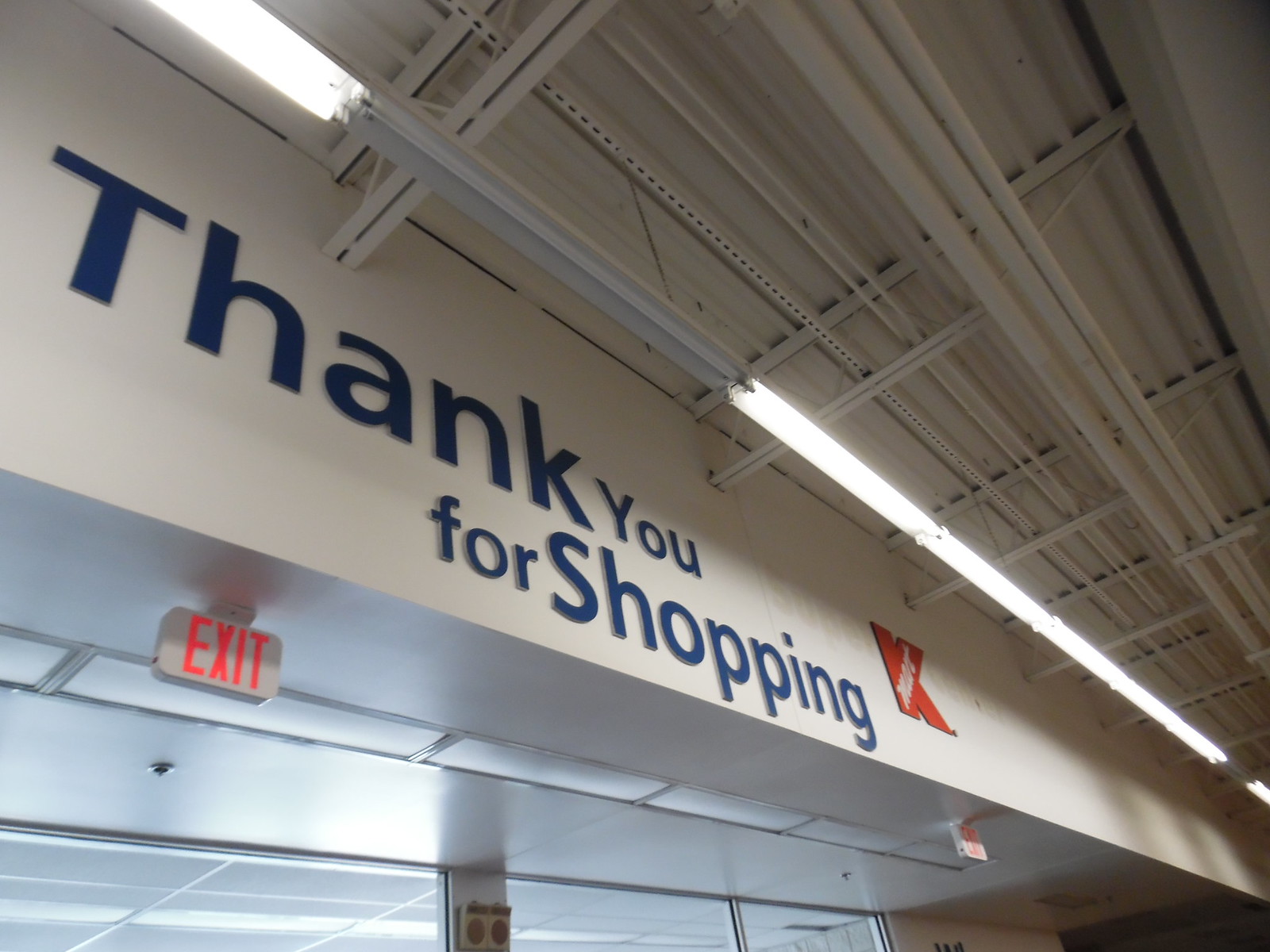This photograph, taken inside a Kmart, captures an upward perspective from the ground level. Dominating the image is a Kmart logo located towards the bottom right corner, featuring a prominent red 'K' with diagonal white lettering likely spelling 'Mart.' The backdrop includes a partial view of glass exit doors positioned in the bottom left corner of the frame, above which a white wall displays blue lettering spelling "Thank you for shopping." This text appears to be affixed to the wall, not painted. Adjacent to this phrase, an illuminated exit sign with red lettering and a white background can be seen mounted on a concrete overhang. The ceiling is populated with long, fluorescent light fixtures, some of which are obscured by the bright lighting. Metal beams and white piping further structure the ceiling area, adding to the industrial feel of the space. Additionally, there is a small fixture protruding from the ceiling that could be a security camera or a sprinkler. This detailed view highlights the architectural elements and signage typical of a Kmart interior.